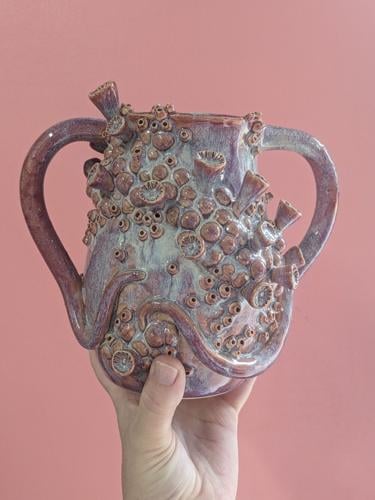In this professional photograph, set against a solid mauve background, a man's hand emerges from the bottom to hold up a striking ceramic vase. The vase, approximately six inches tall, showcases a unique blend of mottled lavender, light gray, and soft blue glaze, giving it an aged appearance. Its form is distinct, with a narrow neck broadening into a bulbous base. Two elaborate handles, reminiscent of curling octopus tentacles, extend from the top and spiral inward, embracing the vase. The surface is richly textured with numerous barnacle-like bumps and circular designs that run diagonally from the top left to the bottom right, offering a 3D coral reef-like aesthetic. These barnacles share the same color palette as the vase, creating a cohesive and visually captivating piece that blurs the line between natural forms and artistic craftsmanship.